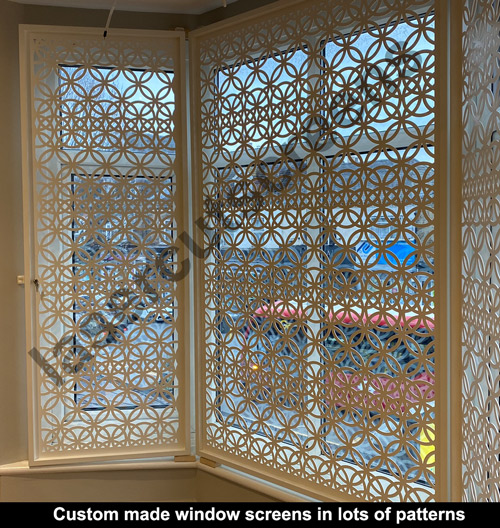This indoor, daylight photograph features a large bay window with a custom-made privacy screen installed within the window assembly. The screen is white, composed of three interconnected parts: a large central rectangle flanked by two smaller rectangles, all joined by folds that likely allow the screen to be folded. The white metal frame holds an intricate pattern of loosely overlapping circles, which partially obscure the view while still letting sunlight through. The window itself is set in a beige wall and through the screen, a red vehicle and a building across the street are faintly visible. Diagonally across the image, gray text reads "Laser Cut Screens," and at the bottom, a black horizontal band features white text stating, "Custom-made window screens in lots of patterns."